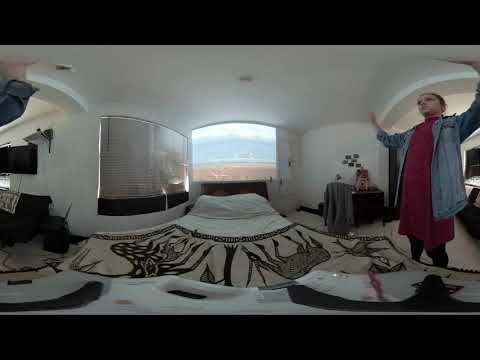This is a detailed panoramic image of a bright, white-walled bedroom captured during the daytime. Dominating the scene is an unmade bed situated in the center, which features white sheets and pillowcases, alongside a lighter brown blanket adorned with detailed black illustrations of various animals, including horses, deer, antelope, and possibly zebras. The bed's blanket, with its intricate design, seems to be partially thrown on the floor.

Behind the bed, there's a large window that floods the room with natural light, displaying an idyllic view of a field and a distant snow-capped mountain. Fluffy white clouds punctuate the blue sky, confirming the daylight setting. To the left of this primary window is another window equipped with closed horizontal blinds and a black ledge.

On the right side of the image stands a Caucasian woman, possibly young, dressed in a distinct outfit: a red dress over black tights, complemented by a light blue denim shirt. Her arms are raised parallel to her head, giving an impression of being held up or perhaps holding the ceiling, adding an intriguing element to the photograph. A special effect or panoramic stitching might give the appearance of her hand reappearing on the opposite side of the room. 

Additional details in the room include a black table and chair with a jacket draped over it, situated to the right. A large glass shelf with a black box at its base can also be seen near the bed, contributing further to the room's decor.